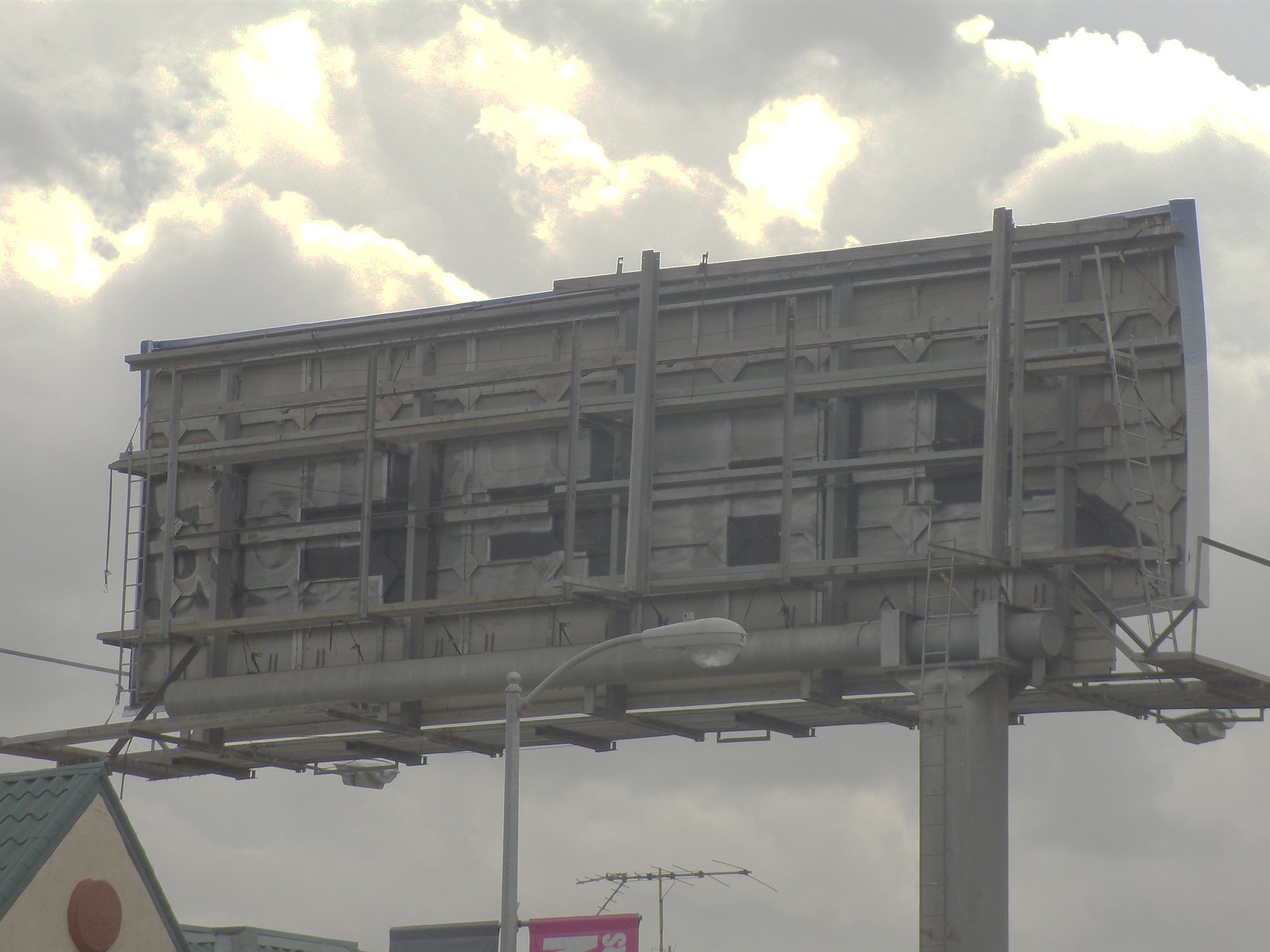This color photograph, taken outdoors, prominently features the gray, metallic back of a billboard, complete with three vertical and numerous horizontal beams. The billboard is mounted on a tall steel pole, which extends down towards the bottom of the image. To the left, you can see the tip of a small building with a V-shaped, triangular roof. The building has a distinctive blue roof, a tan front, and a round, light brown circle or icon in the middle of the gable. A gray streetlamp is visible in the foreground, partially obscuring the view. Further in the background, an antenna is situated below the billboard. The sky is filled with gray clouds, with some bright light breaking through, adding an industrial yet atmospheric feel to the scene. Toward the middle of the photo, parts of a red sign and another gray sign are also visible.